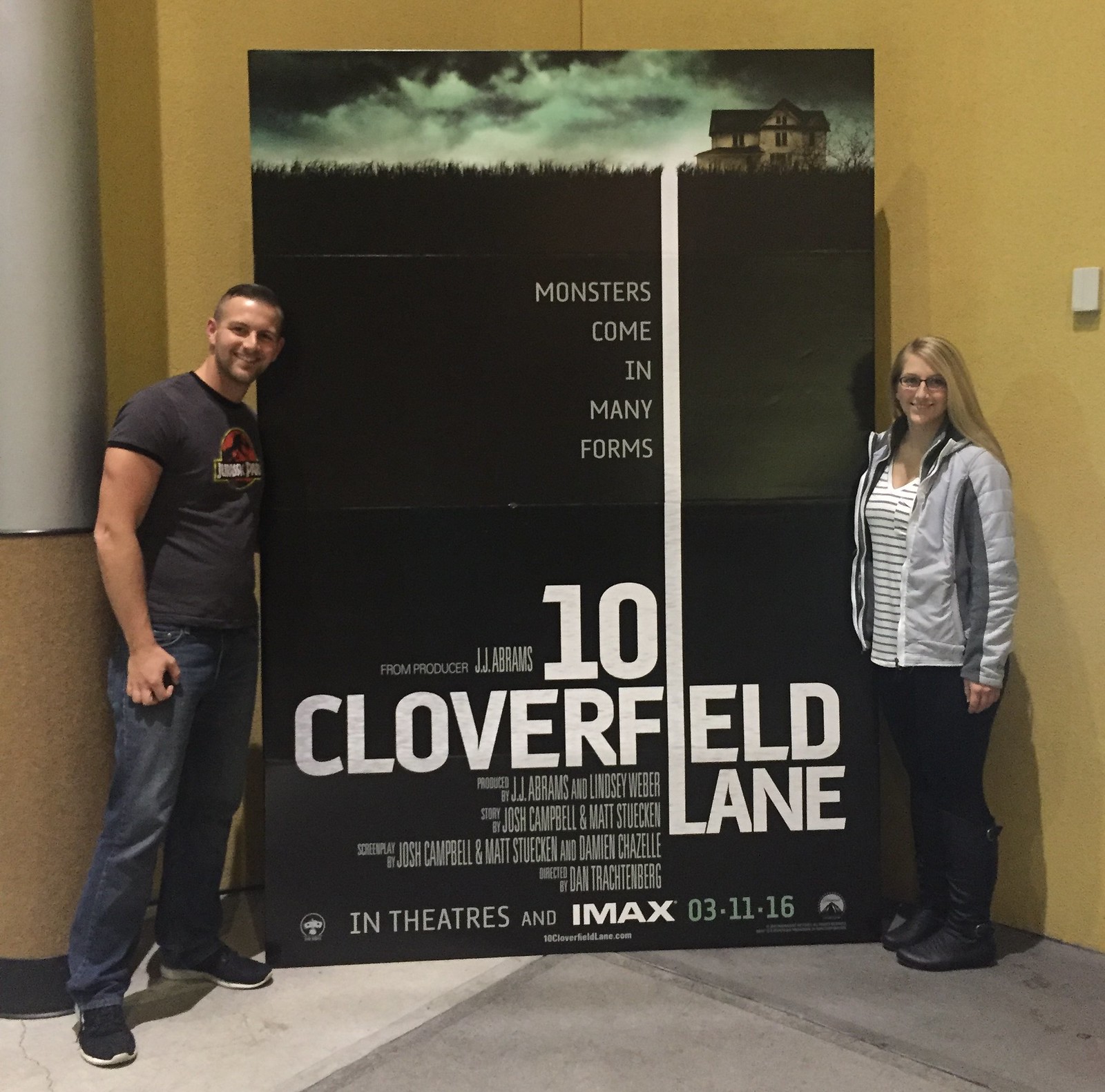The image captures a large square display featuring a man and a woman standing next to an imposing poster for the movie "10 Cloverfield Lane." The background is a simple brown wall, suggesting the photo was taken indoors, likely at a movie theater. The man, positioned to the left of the poster, has short brown hair and thin facial hair. He is casually dressed in a dark gray, short-sleeved Jurassic Park t-shirt, jeans, and black tennis shoes. The woman, standing to the right, sports a blonde hairstyle, glasses, and is clothed in a gray jacket over a white and blue striped shirt, paired with black pants and tall black boots. Both individuals are smiling happily at the camera.

The centerpiece, a tall cardboard promotional display for "10 Cloverfield Lane," has an upper portion depicting a haunting nighttime sky with white and green-tinged clouds, a sinister-looking house, and grass, amidst which the phrase "MONSTERS COME IN MANY FORMS" is right-aligned in white, all-capital letters. The main body of the poster is solid black, listing the film’s title "10 Cloverfield Lane" in large white text at the bottom, along with the names of the cast, director, and producers right-aligned below it. The release date, "In theaters and IMAX 03-11-16," is prominently displayed at the very bottom, completing the striking promotional exhibit.